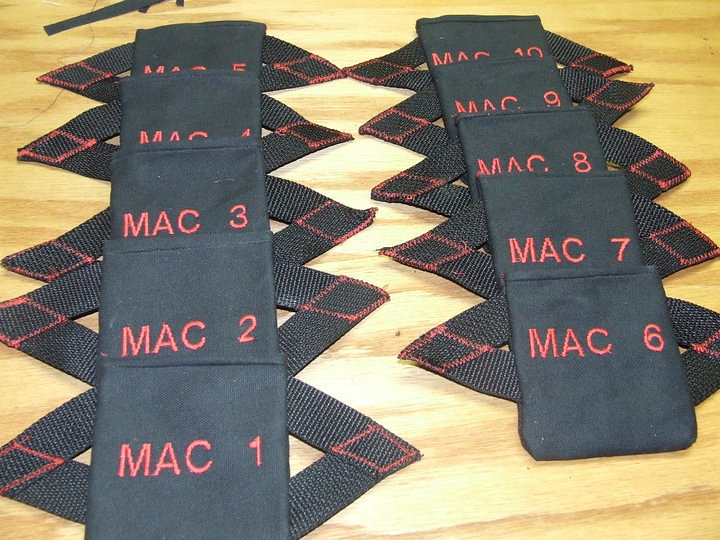The image displays two columns of black rectangular fabric pieces stacked slightly on top of each other, arranged vertically on a wooden surface that has a yellowish-gray tint. Each piece features the word "MAC" in large, red, capital block letters, followed by a number ranging from 1 to 10. The left column features MAC 1 through MAC 5 from bottom to top, while the right column features MAC 6 through MAC 10 in the same order. The fabric pieces include black triangular extensions on both sides, with red diamond patterns knitted into the upper part of each triangle.